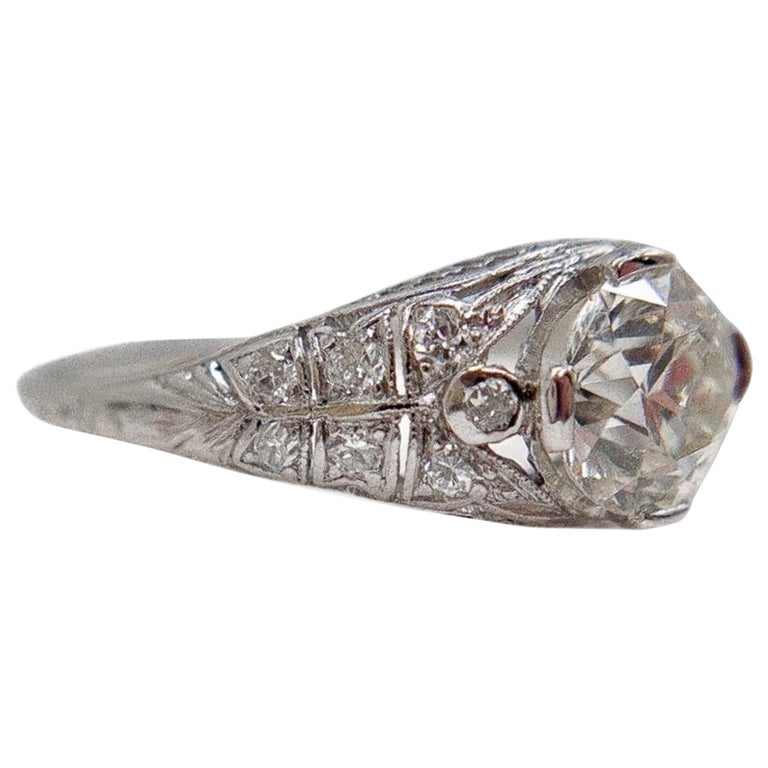This is a detailed close-up photograph of what appears to be a ring, although the exact perspective makes it somewhat ambiguous. The primary element in focus is a large gemstone, which is likely a rose-cut diamond, embedded on the right side of the ring as viewed. The setting appears to be made of a silvery metal, possibly platinum, and the stone is secured by four prongs at the top, sides, and bottom. The band tapers towards the back and features intricate detail work, including a pattern with a smaller diamond mounted just below the main stone.

On the visible side of the band, there are additional smaller diamonds arranged in a decorative design. This includes round diamonds closest to the main gemstone, followed by a section with almost square, artistically cut diamonds in a square setting. The artistry extends to facets cut into the ring right below these smaller diamonds, suggesting a notable level of craftsmanship.

The ring lies flat on an unseen surface with no background to distract from its detailed design. The foreground, particularly the area around the main diamond, is in sharp focus, while the other parts of the band and details are slightly blurred, drawing attention to the intricacy of the gemstone and its surrounding settings.